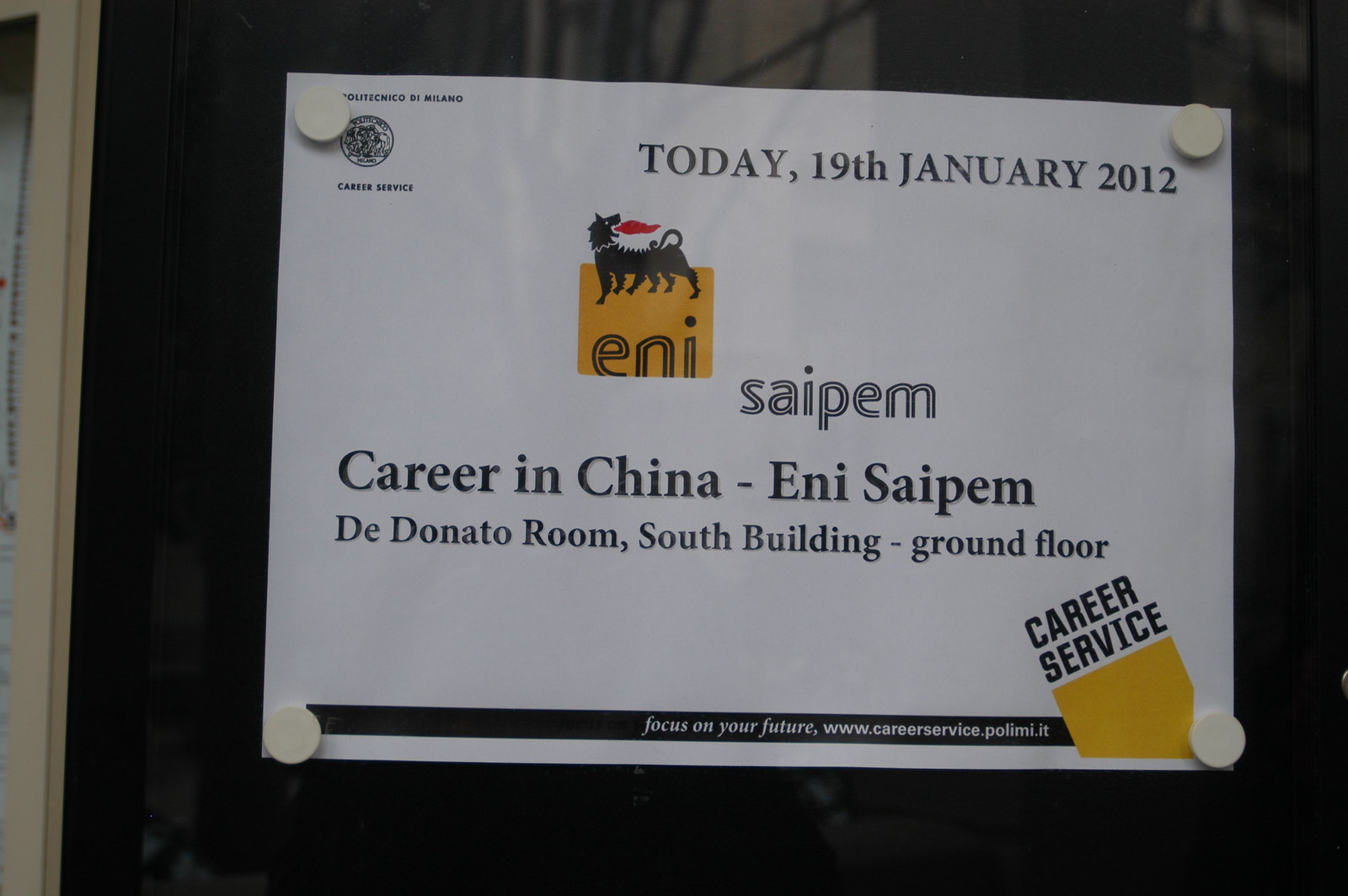The photograph captures an 8.5 x 11 inch white sign held up by four round magnets, one at each corner, adhered to a window, possibly belonging to a business or office building. The sign prominently displays the date "Today, 19th January 2012" at the top, along with the ENI SAIPEM logo, which features an animal resembling a dragon or creature breathing fire. The text on the sign announces a career services event titled "Career in China - ENI SAIPEM" to be held at the Donata Room, South Building, ground floor. Additionally, the sign notes a website link, www.careerservice.palemmi.it. The bottom of the sign features a blue line with the slogan "Focus on your future," and in the lower right-hand corner, there is another career service logo with a yellow portion beneath it. The sign's text is in black or blue.